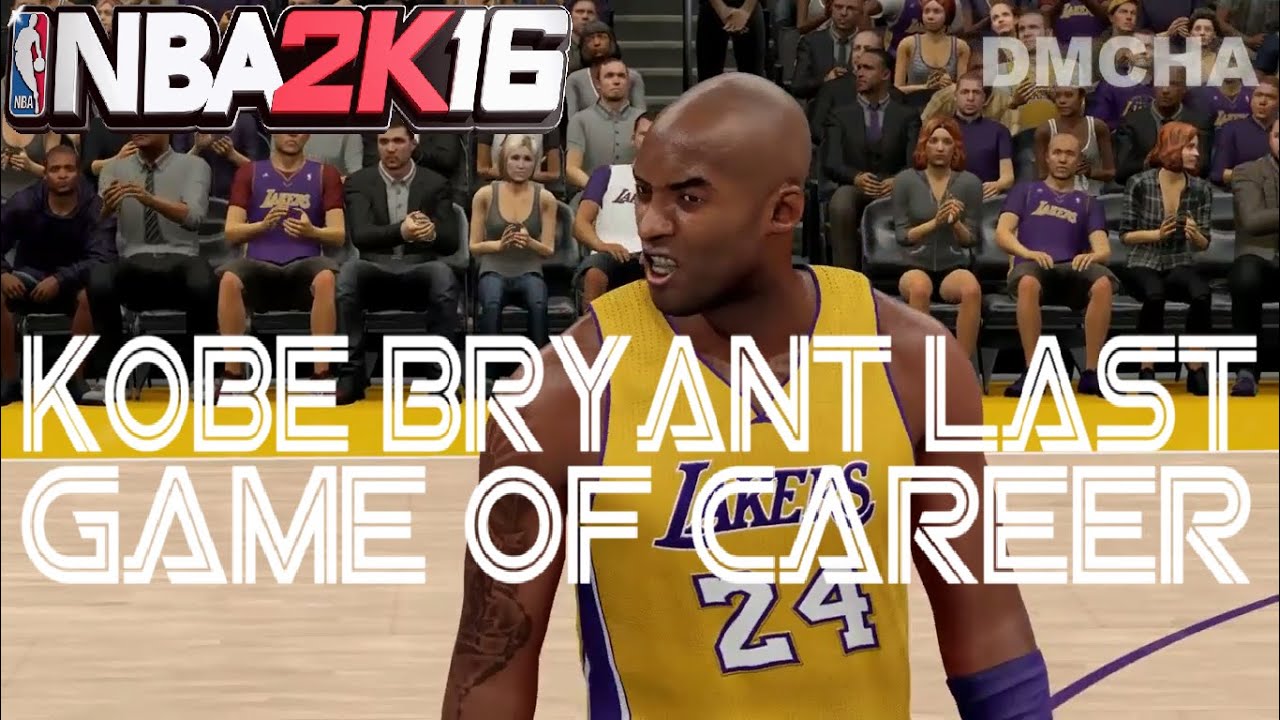The image portrays the cover of the video game NBA 2K16, specifically highlighting a special edition titled "Kobe Bryant: Last Game of Career." Dominating the center is a close-up depiction of Kobe Bryant rendered in the game's realistic graphics. Kobe is captured mid-action with a determined scowl on his face, reflecting his intense focus and competitive spirit. The background showcases a blurred sea of fans in the stands, many adorned in purple shirts and Los Angeles Lakers attire, energetically clapping and celebrating the legendary player's illustrious career. The visual composition powerfully encapsulates the emotion and grandeur of Kobe Bryant's final moments on the court.